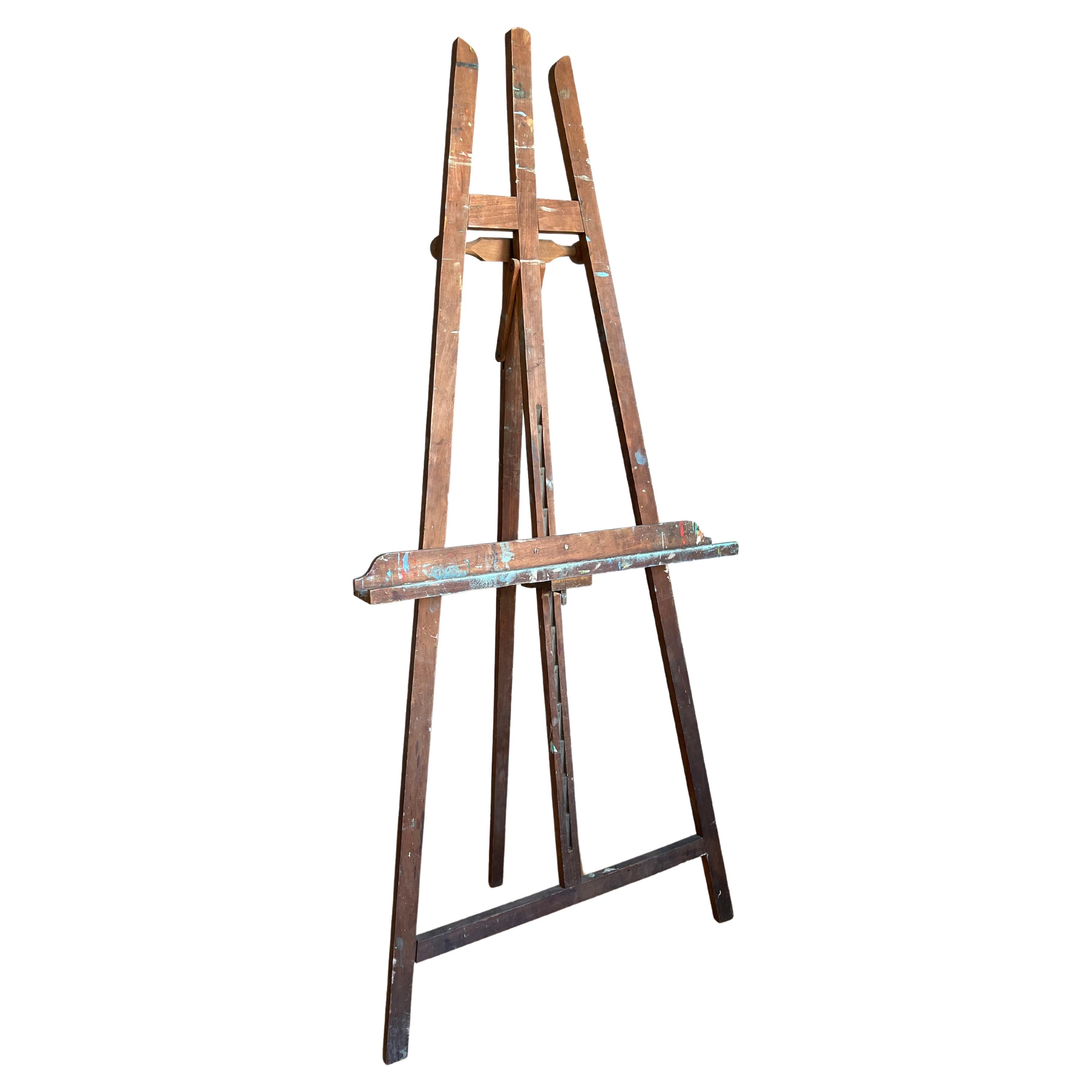The image features a tall, well-used wooden art easel set against a solid white background. The easel is a traditional three-legged design, with two front legs and a single back leg extending out for support, creating a stable triangular frame. The wood appears aged with nicks, and there are noticeable paint splatters, predominantly blue and green, indicating extensive use. A central vertical slat runs from the top to the bottom, where it connects to a wooden brace. The horizontal shelf in the middle, designed to hold the painting canvas, has visible blue paint marks. The easel is adjustable, with slots allowing the base to raise or lower to accommodate various canvas sizes, and it can be folded flat for convenience. The overall impression is of a well-loved and frequently used artist’s tool, ready for the next creative project.